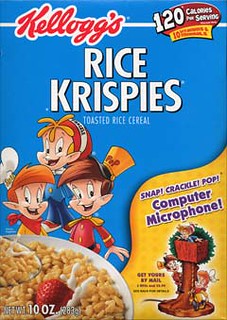This detailed portrait image showcases an old Kellogg's Rice Krispies cereal box with a distinct blue background. In the upper left-hand corner, the iconic Kellogg's logo is written in red cursive. To its right, a red bubble contains white text indicating "120 calories per serving." Dominating the center of the box, "Rice Krispies" is prominently displayed in large white uppercase letters, with the phrase "Toasted Rice Cereal" in smaller print just below. The three familiar Rice Krispies mascots—Snap, Crackle, and Pop—dressed in their characteristic colorful outfits (one in a chef's hat, another in a yellow rectangular hat) are cheerfully grouped near the middle left side. On the lower left, a cut-off bowl of Rice Krispies with a spoon and a strawberry is visible. The lower right corner features a yellow background with purple text that reads "Snap, Crackle, Pop, computer microphone, get yours by mail." In this section, the three mascots are illustrated around a mailbox, enhancing the nostalgia of the vintage packaging. At the very bottom left, the box indicates a net weight of 10 ounces.